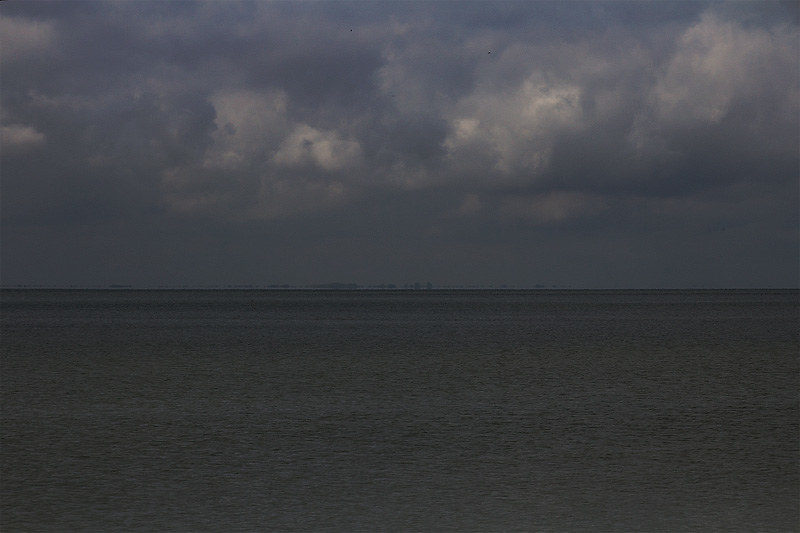This photograph captures a dimly lit ocean scene, possibly taken during dusk or amidst an approaching storm. The bottom half of the image shows a body of water, almost black in appearance, with subtle ripples and a cold, choppy texture. The upper half of the image features a nearly overcast sky filled with large, fluffy clouds in varying shades of gray and white. The horizon line is strikingly straight and even, blending seamlessly with the sky above. In the distant background, barely discernible, are tiny structures resembling buildings, hinting at a distant shoreline or cityscape. Overall, the image conveys a somber and foreboding maritime atmosphere.